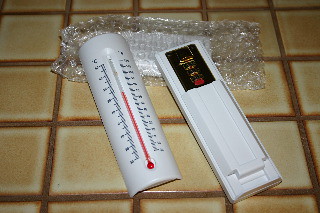A newly purchased white thermometer, clearly just taken out of its packaging, rests on what appears to be a tiled countertop. This assumption is based on the presence of small, approximately 2x2 inch brown tiles with darker brown grout lines characteristic of a countertop rather than a floor. The thermometer, still accompanied by the bubble wrap it came in, consists of two interlocking parts: a flat base, presumably meant to be affixed to a wall, and a rounded piece that houses the actual temperature reading mechanism. This allows for sliding the thermometer on and off the base. Temperature measurements are displayed in both Celsius (left) and Fahrenheit (right). The thermometer indicates a temperature about three-fourths up the readable scale, though the exact temperature is indiscernible because the text is blurry. The entire setup, including the bubble wrap, is visible on the countertop.